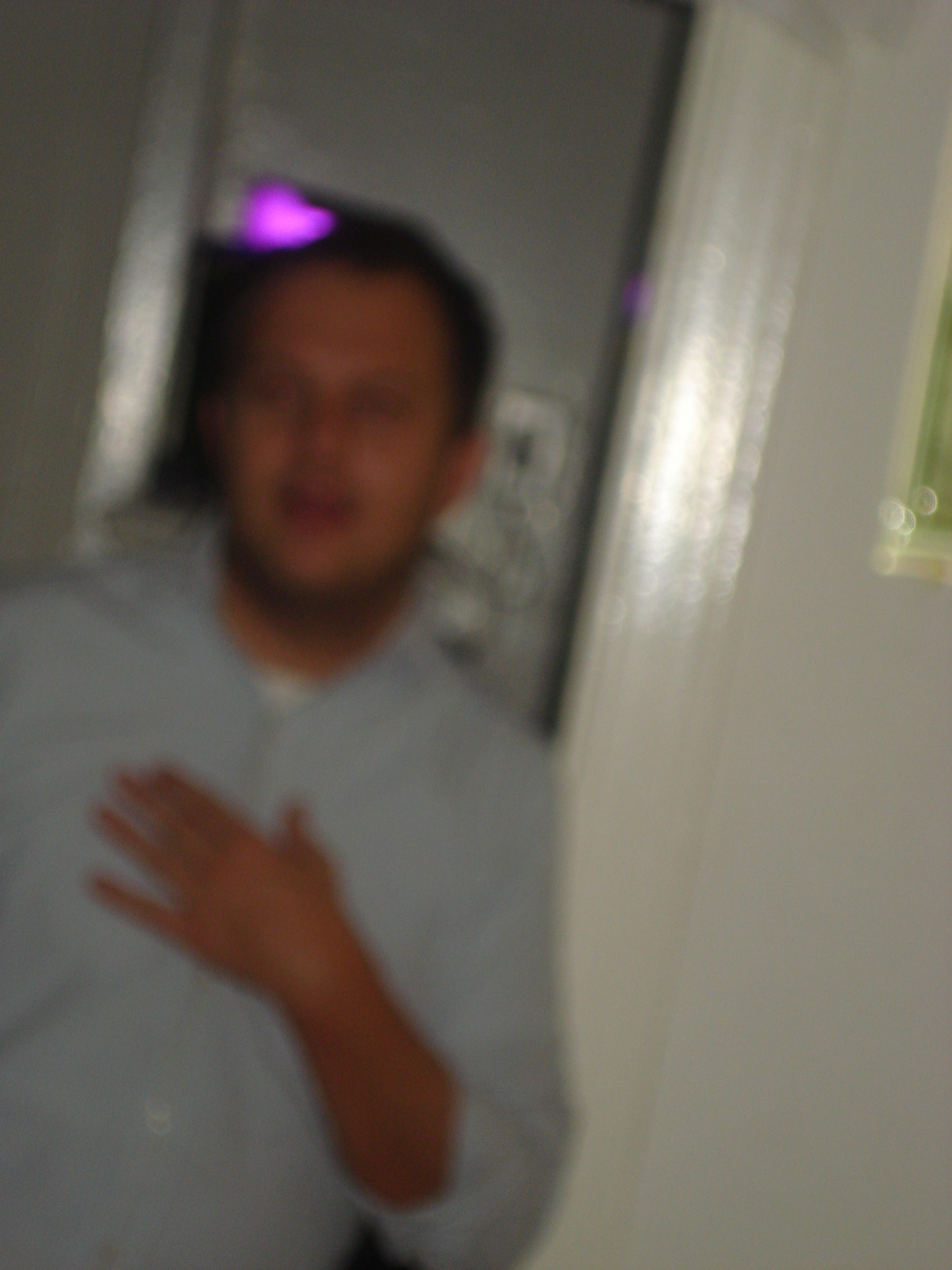This is a close-up and blurred portrait photograph of a young Caucasian man, likely in his teens, 20s, or 30s, standing in a hallway lined with white walls and a white, reflective door frame. Dressed in a light blue short-sleeve dress shirt with a white undershirt, his white shirt buttons are visible. The right sleeve of his shirt is rolled up, showing a large portion of his left forearm. He has light skin, short brown hair, and a brown beard and mustache. His right hand is placed over his left breast, his expression suggesting surprise or contemplation, with his mouth slightly open. His face is blurred, obscuring detailed features. Behind him, the door frame reveals a white wall with some blurred objects and a shiny, purple light above his head, possibly from an electronic control or room lighting. A picture frame with a gold outline and a light green matting is partially visible on the right-hand side of the image.